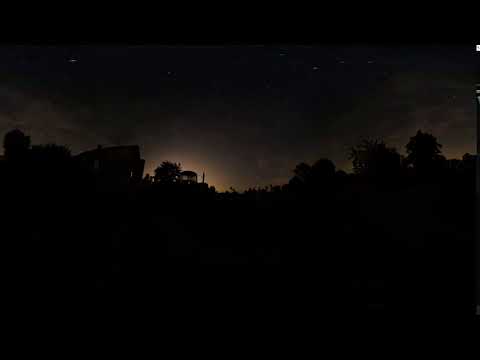This is a detailed night scene image. The bottom half of the photo is enveloped in darkness, with several low buildings and trees silhouetted against a subtly backlit sky. The sky itself reveals a mesmerizing mix of hazy, diffused clouds stretching from center-left to the right, gradually transitioning to a rich purple hue as you move upward. Scattered stars pepper the sky, offering a glimpse into the cosmos above. At the center-left portion of the image, a low glow, possibly from a setting sun or an artificial light source, creates an ethereal illumination behind a larger building and some trees. The silhouettes dip towards the center and rise towards the edges, suggesting the presence of gentle hills or varying terrain. Additionally, there might be a pole or tower faintly visible at the center, contributing to the night’s intricate tapestry. The overwhelming darkness of the scene adds a sense of depth and mystery, drawing attention to the subtle details illuminated in the lower horizon.